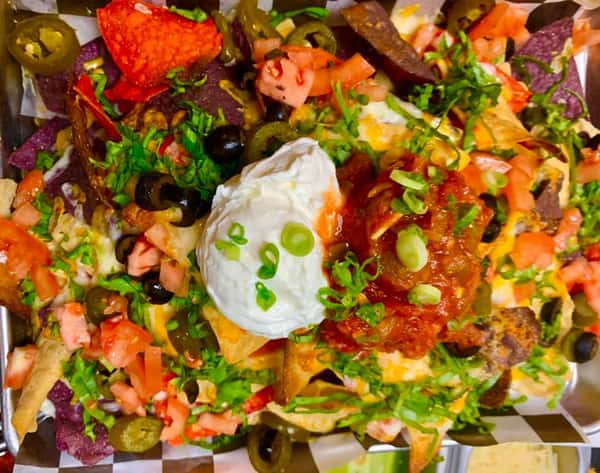In this vibrant and enticing close-up of a loaded nacho dish, a box lined with checkered paper cradles a colorful feast. The photograph, taken from a top-down perspective, offers a detailed view of the nachos, which are adorned with an array of toppings. Dominating the center are dollops of creamy white sour cream to the left and bright red salsa to the right, both sprinkled with finely chopped green onions. The nachos themselves are a mix of multicolored chips—yellow, red, purple, and brown—providing a visually appealing foundation.

Scattered throughout the dish are sliced habanero peppers and chives, adding vibrant green and red accents. Melted cheese weaves through the layers of chips, while bits of tomatoes and olives are nestled within, contributing to the rich tapestry of flavors and colors. Despite the abundance of vegetables and cheese, there is no visible meat, suggesting this might be a vegetarian rendition of the popular snack. The black and white checkered paper lining not only enhances the presentation but also prevents the food from staining the box, reinforcing both style and practicality in this delightful example of food photography.